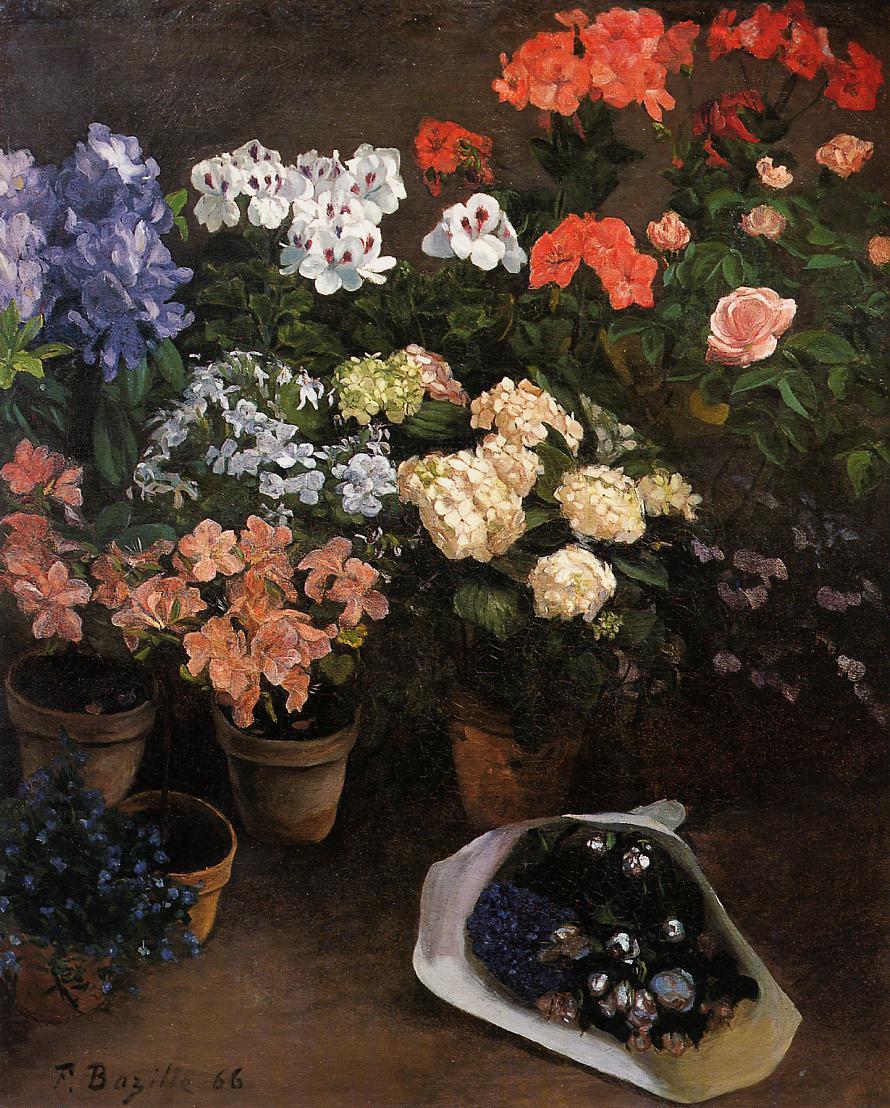The painting is a detailed and vivid depiction of a collection of potted flowers set against a brown background. Various terracotta pots in the scene hold a wide array of flowers including yellow, pink, blue, red, white with black dots, and bluish-purple irises. Notably, light pink roses can be seen on the right side. Towards the bottom right corner, a bouquet wrapped in white paper lies on the ground, containing blue, white, light blue, and pink flowers. The artwork is signed in the bottom left corner by the artist, P. Bazille, with the number '66. The scene is realistically rendered, showcasing flowers of multiple colors, shapes, and sizes, with some pots in the background contributing to the depth of the composition.